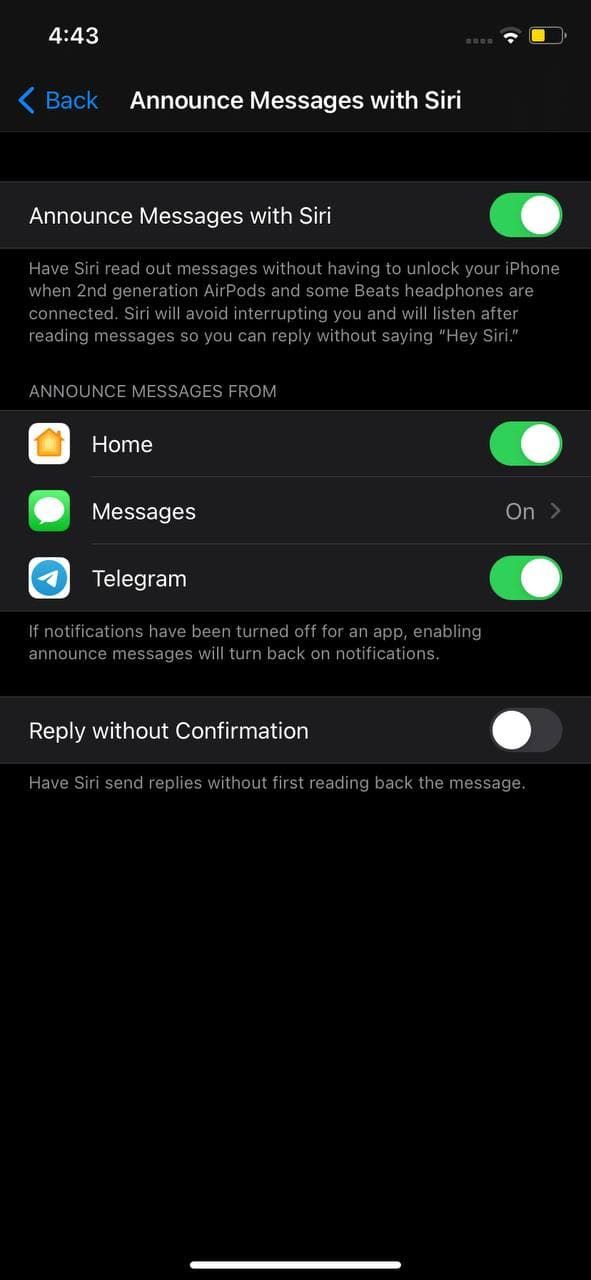The image is a detailed screenshot of an iPhone's settings specifically related to Siri. In the status bar at the top right corner, the battery icon indicates the battery level is approximately 30% and the color is yellow, implying low power mode. To the left of the battery icon, the Wi-Fi signal shows two out of three bars, suggesting a moderate Wi-Fi connection. Next to the Wi-Fi icon, there are four light gray dots.

On the top left of the screenshot, the current time is displayed in white text as 4:43. Centrally, the title "Announce Messages with Siri" can be seen, with a blue "Back" option accompanied by a leftward arrow to its left.

Below this header, the option "Announce Messages with Siri" is written in white text with a green toggle switch turned on. Underneath this section, there are three categories listed: "Home," "Messages," and "Telegram." To the right of "Home" and "Telegram," the green toggle switches are both turned on. However, next to "Messages," instead of a toggle switch, the word "On" and an arrow pointing to the right are displayed.